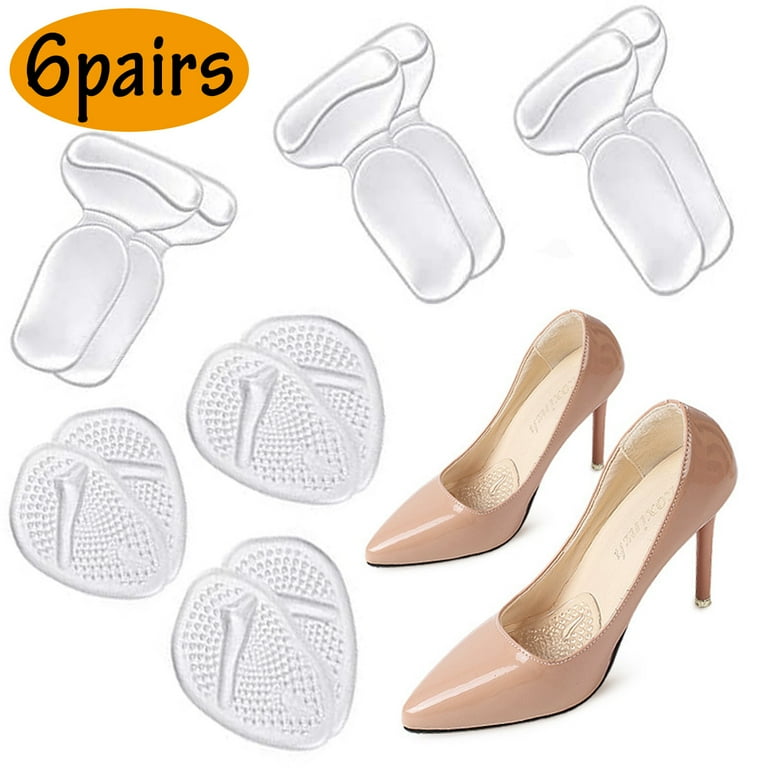This professional advertisement showcases translucent gel inserts designed for high-heeled women’s shoes against a crisp white studio background. In the top left corner, there is an orange oval with black text reading "6 pairs," indicating the quantity of inserts available. The image features two different types of inserts: the top row has three inserts shaped similar to a razor with a wider top and narrower bottom, suggesting they fit the ball of the foot, while the lower left corner displays three inserts in an uneven elliptical shape, presumably for the heel. These inserts are arranged in a triangular formation. A pair of stylish high-heeled shoes, in a light pinkish-salmon color with a narrow stiletto heel and light yellow lining, is showcased on the lower right corner, displaying the clear gel pads comfortably placed inside, highlighting their function as anti-slip and cushioning aids. The patent leather-like finish of the shoes adds a refined touch to the overall advertisement, emphasizing both style and functionality.